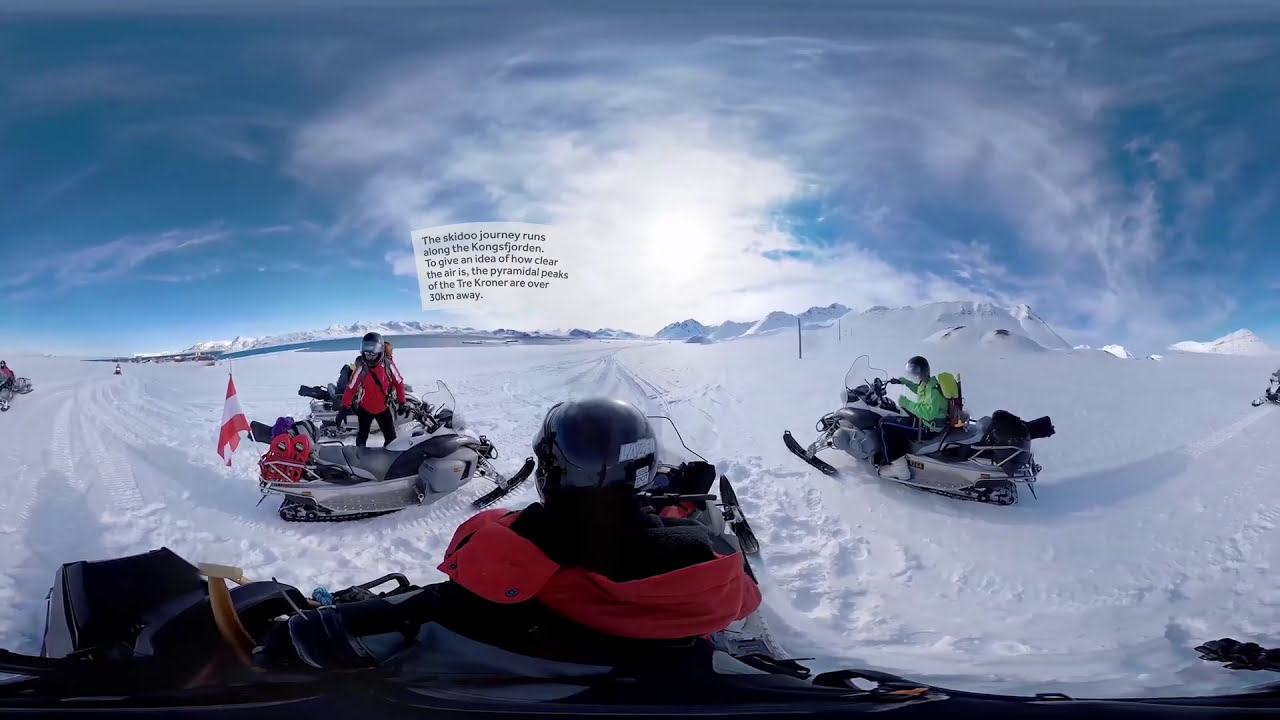In this vibrant daytime photograph, we see three individuals navigating a vast, snow-covered landscape under a brilliant blue sky with swirly clouds and a bright white sun at its center, contributing to the cold ambiance. The bottom portion of the image features the upper half of a snowmobiler facing away from us, with a black helmet and a black and red coat. To the left is another individual on a gray snowmobile, identifiable by their red jacket and the red and white flag affixed to the back of their vehicle. The right side displays yet another snowmobiler, distinguished by their green jacket and yellow backpack, riding a gray snowmobile facing left. Notably, there's a slight wavy effect to the image, likely due to the virtual reality nature of the shot, creating a surreal, almost warped appearance in both the snow and sky. Hovering near the sun, a white square with black print provides a detail about the location, mentioning the "Ski-Doo Journey running along the Kongsfjorden," with the sharp peaks of the Trey-Kroner visible some 30 kilometers away, showcasing the clarity of the frigid air.